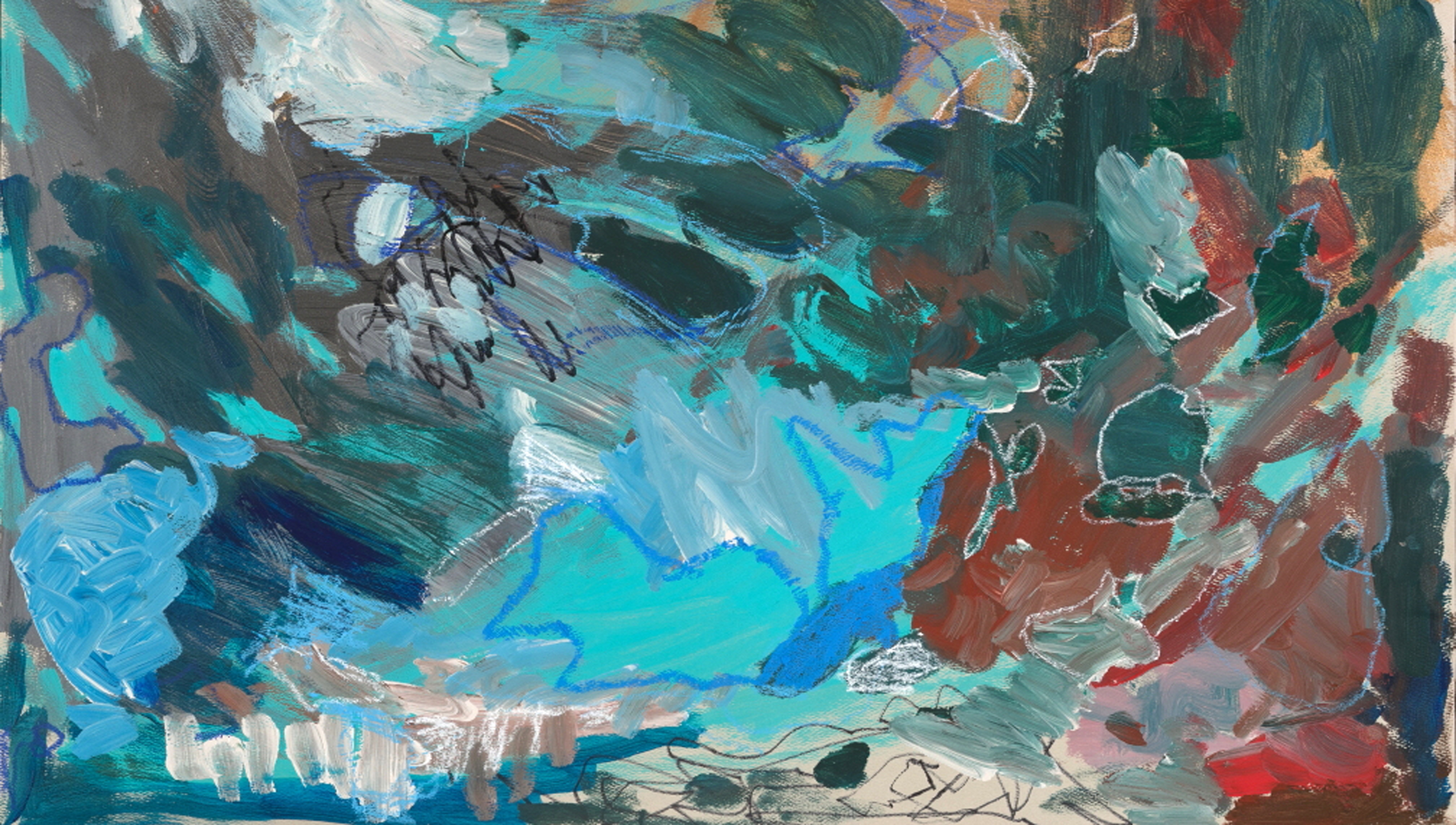This is a dynamic and completely abstract oil painting featuring an explosion of multicolored brushstrokes that create a complex and intriguing composition. Predominantly using dark blues, grays, and medium blues, the artwork also incorporates vibrant splashes of red, baby blue, teal, dark gray, green, orange, dark red, brown, and white. The seemingly random brushstrokes merge to form an intricate pattern, with certain areas resembling various objects, though they remain highly ambiguous, like in a Rorschach test. Towards the right, the hues of red-gray and red might suggest the form of a character, a tree, a log, or possibly an animal's head. On the left, cloud-like shapes fade into the background. The painting features wide, sweeping strokes, occasionally layered on top of each other. Post-drying, the artist appears to have used white chalk to trace around approximately 10 to 12 different shapes, adding another layer of abstraction. A black line drawing at the bottom adds further complexity, enhancing the enigmatic and underwater-like feel of the painting. The artist’s signature, inked in the middle, punctuates the composition, cementing it as a deeply engaging and surreal visual experience.